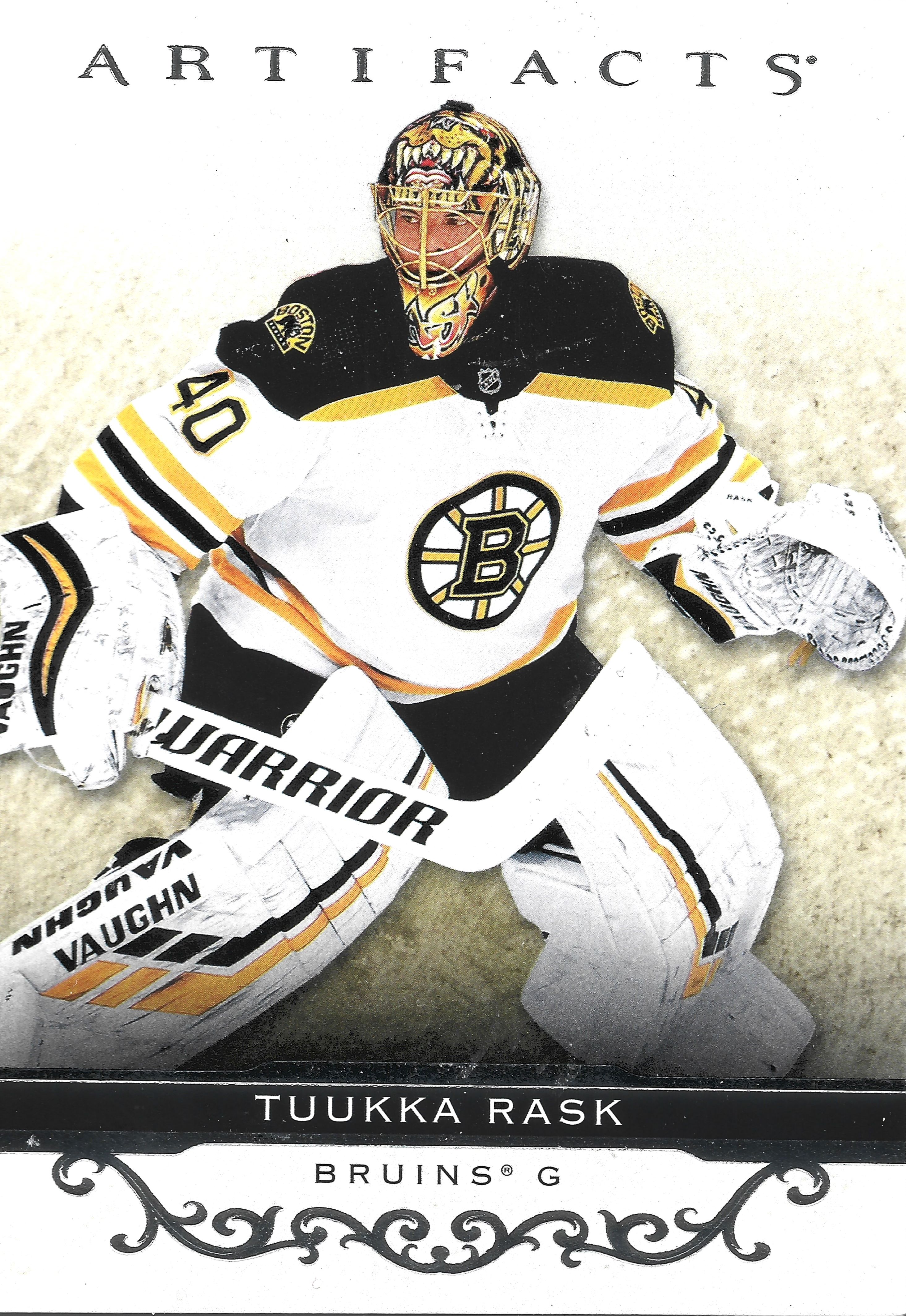This is an image of a hockey card featuring Tuka Rask, a player from the Bruins. The card's background is predominantly white with hints of gray, and at the top, it displays the word "Artifacts" in black writing. Tuka Rask is pictured wearing full hockey gear, including a black helmet adorned with animal fangs in beige and white, a chin guard, and protective padding. His jersey is black at the top with a gold bar, transitions to white at the body, and features a prominent letter "B" in a circle in the center, surrounded by yellow, black, and orange stripes on the sleeves. His white mittens and white Warrior-branded hockey stick complement his ensemble. He also wears black pants with white leg guards and additional padding over his arms and legs. At the bottom of the card, a black bar with white writing displays "Tuka Rask," and below that, "Bruins G" is written in black on a white background. Additionally, the card includes a fancy floral vine frame at the bottom.